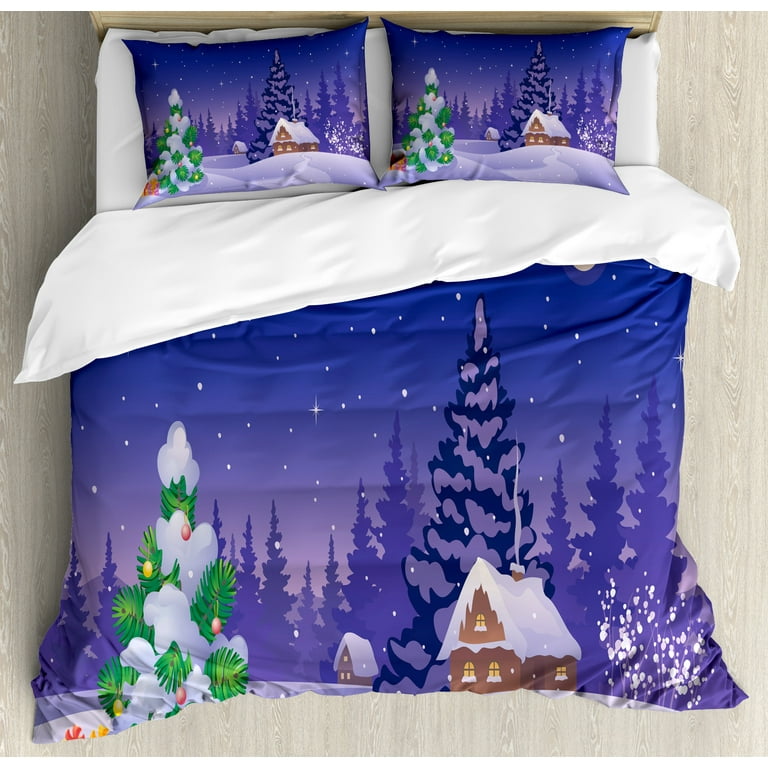This photograph depicts a beautifully styled bed set, perfect for the holiday season. The bed features a winter-themed comforter and matching pillowcases, all showcasing a vibrant Christmas scene. The comforter and pillows depict a night sky with white stars and gently falling snowflakes. The lower part of the comforter is adorned with silhouetted evergreen trees in shades of purple and lavender, transitioning into a serene blue sky. 

A snow-covered Christmas tree with green branches and colorful ornaments stands prominently on the left, while on the right, there is a tall, deep purple pine tree also laden with snow. Nestled between the trees, there are two cozy, snow-clad cabins with lit windows, one adorned with a chimney. The detailed design on the bedding seamlessly extends to the pillowcases, echoing the same enchanting scene. The backdrop of the image features a tan wood headboard and a grayish wood wall, complementing the light-colored wood floor seen around the bed. The underside of the comforter is a crisp white, matching the white sheets beneath it, completing the festive yet cozy ensemble.